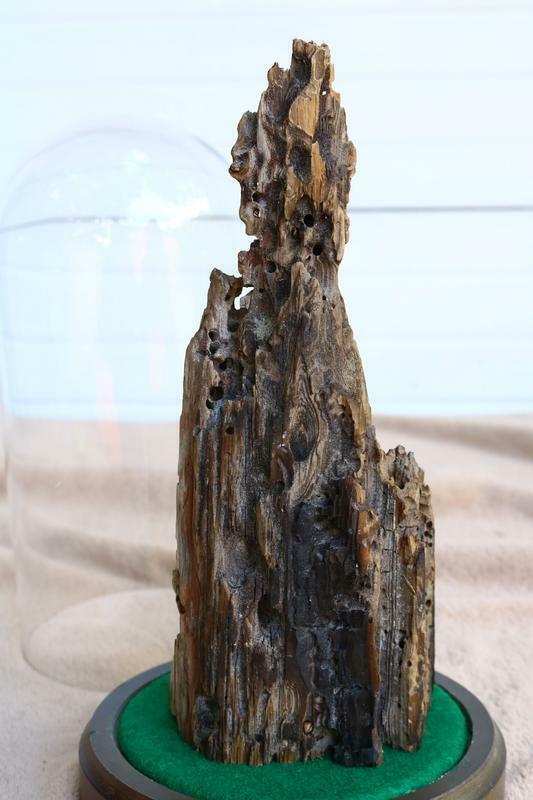The photograph showcases what appears to be a jagged, vertical piece of fossilized or petrified wood. This striking structure, which narrows to a point at the top, stands on a green felt surface that covers a circular brown wooden base. The wood, marked by grain patterns, knot holes, and possible insect or worm damage, displays a range of brown and black hues, enhancing its ancient, weathered appearance. The base rests on light brown sand, adding to the naturalistic presentation. The backdrop features white or possibly light blue wooden planks, which provide a subtle contrast to the earthy tones of the fossilized wood. The image highlights intricate details such as the ridges and holes in the petrified wood, sparking curiosity about its age and origins.